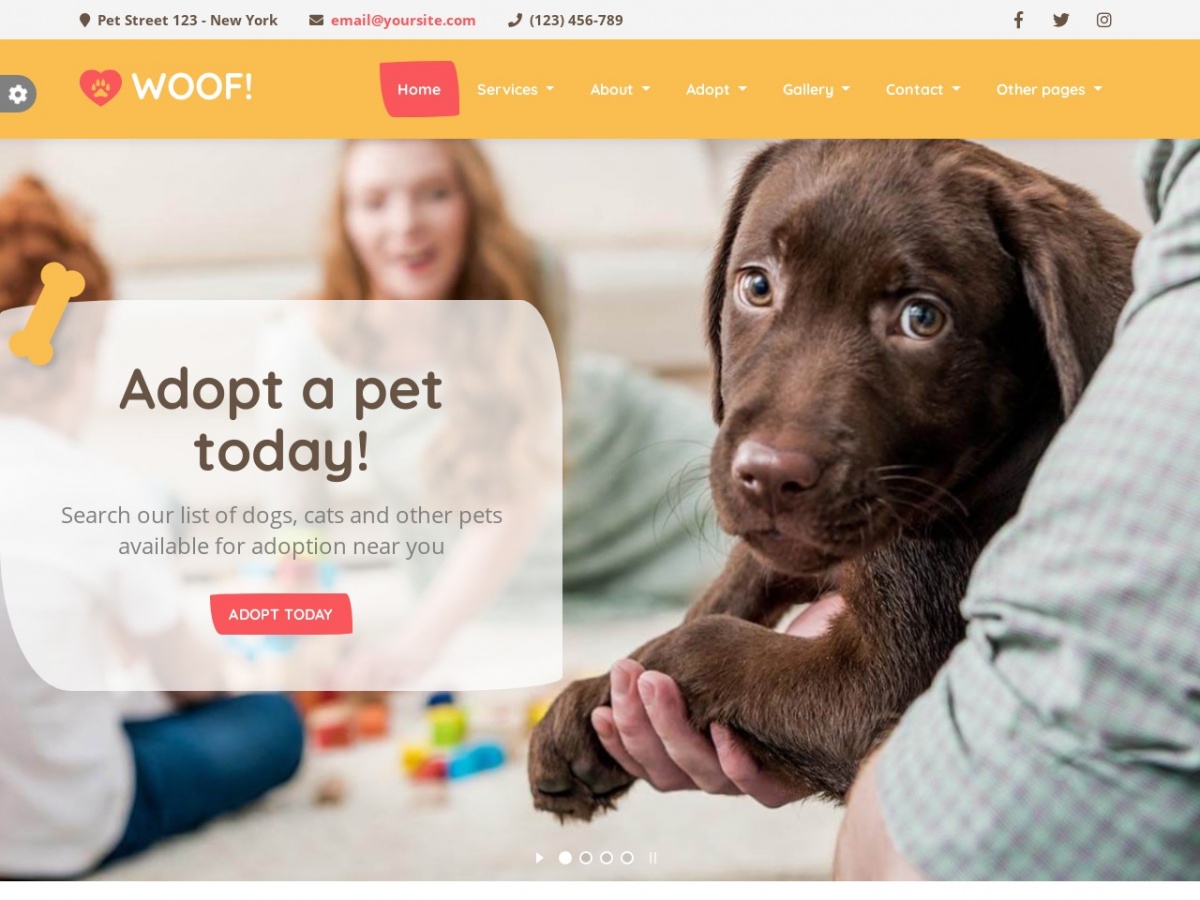This is a detailed and cleaned-up caption for the image described:

---

The image is a screenshot of a website's homepage, predominantly featuring the branding and a call to action for pet adoption. The top menu has a light orange background, with the organization's name, "WOOF!" displayed in white text alongside their logo—a red heart with a light orange dog's paw print. 

Occupying the majority of the webpage is a poignant, close-up photograph of a brown dog with solid brown fur and sorrowful brown eyes, looking directly at the camera. A person's arm, barely visible, holds the dog, adding a sense of comfort to the scene.

Superimposed on the left side of the photo is a semi-transparent large square with the headline, "Adopt a Pet Today!" in bold text. Below that, it reads, "Search our list of dogs, cats, and other pets available for adoption near you." Further down, a red rectangle button with white text invites users to "Adopt Today."

The top menu, from left to right, includes links labeled Home, Services, About, Adopt, Gallery, and Contact. A gray border at the very top of the page displays placeholder text reading "Pet Street 123 - New York" and an email address "email@yoursite.com," indicating that this could be a template for a website.

---

This refined caption provides a clear and detailed description of the website homepage, detailing both its visual elements and design features.